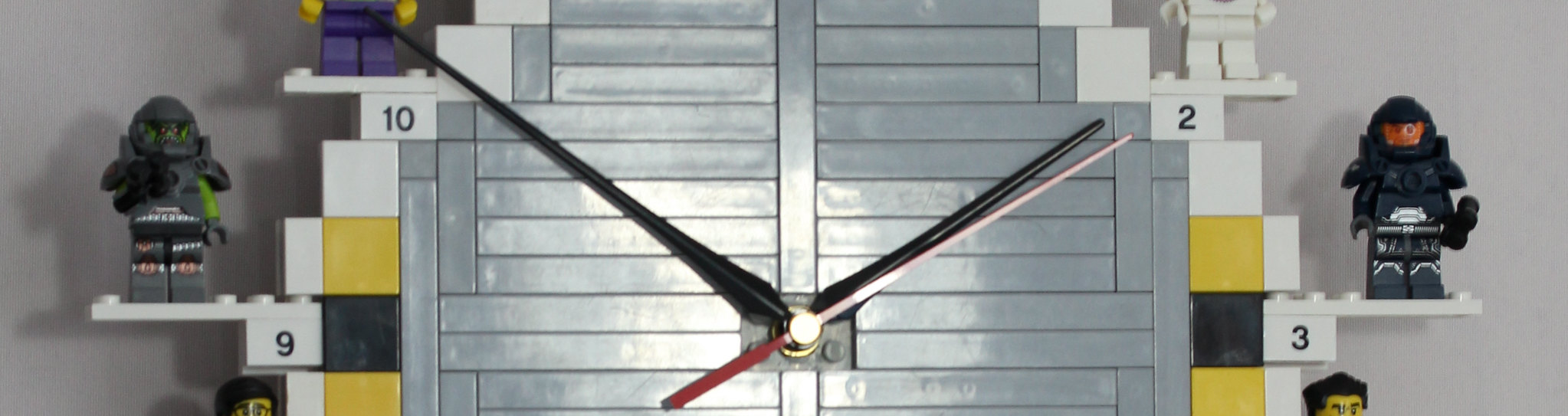This photograph features a close-up of a uniquely designed clock constructed entirely from Lego pieces, set against a light gray wall. The clock face is made of stacked gray rectangular Legos, with black hour and minute hands and a red second hand, currently stopped at 1:52:10. The outer frame of the clock incorporates white, yellow, and black Lego pieces. Notably, there are visible numbers – 2, 3, 9, and 10 – with small ledges protruding from each number. These ledges host Lego figures designed to resemble superheroes or characters, including ones positioned at the 3, 9, and 10, with additional figures just out of view below the numbers 3 and 9. The entire image showcases the intricate detail and creativity involved in this Lego clock construction.